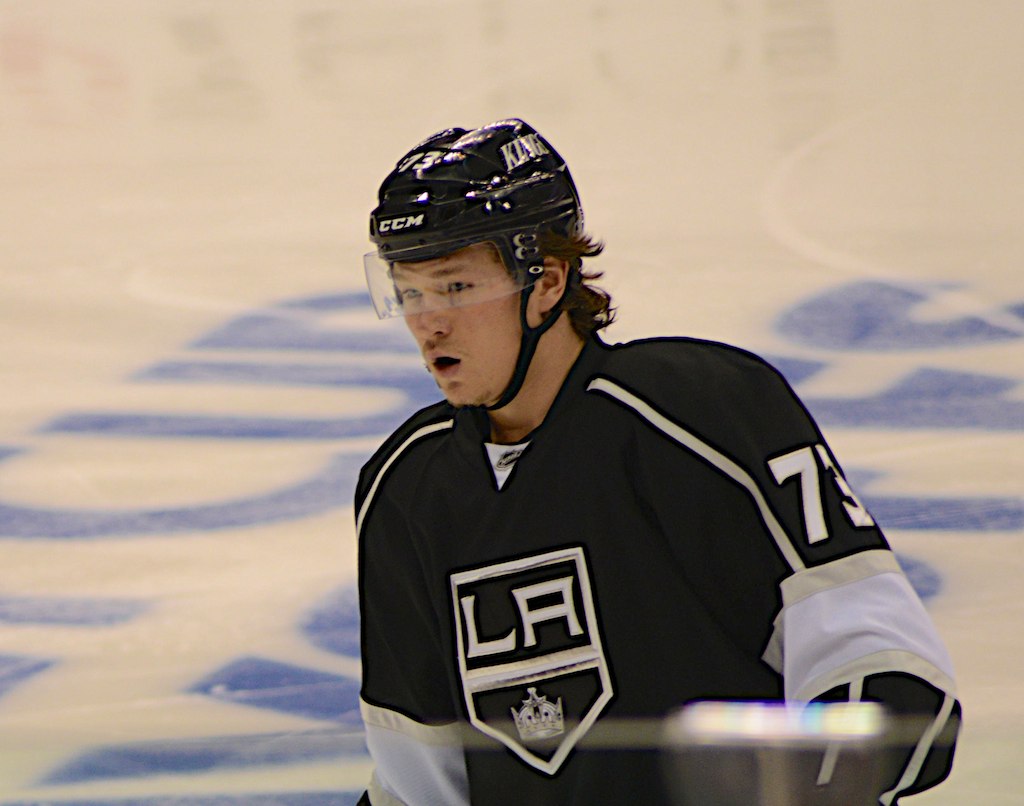This photograph captures a mid-20s, male, Caucasian professional hockey player from the LA Kings, identified as number 73, centered on the ice during a warm-up session. He is framed from the belly button up, wearing a black helmet with a clear visor, marked with "Kings" on the side and "CCM" on the front, along with his number 73 in white. His black jersey features the LA Kings logo, consisting of white "LA" lettering within a half-diamond, half-square shape, accompanied by a crown. The sleeves of his jersey have distinctive white stripes down to the wrists, with white sections around the elbows. The blurry and noisy picture quality, potentially a cropped video screenshot, shows a backdrop of an ice hockey rink with partially visible blue text on the ice.